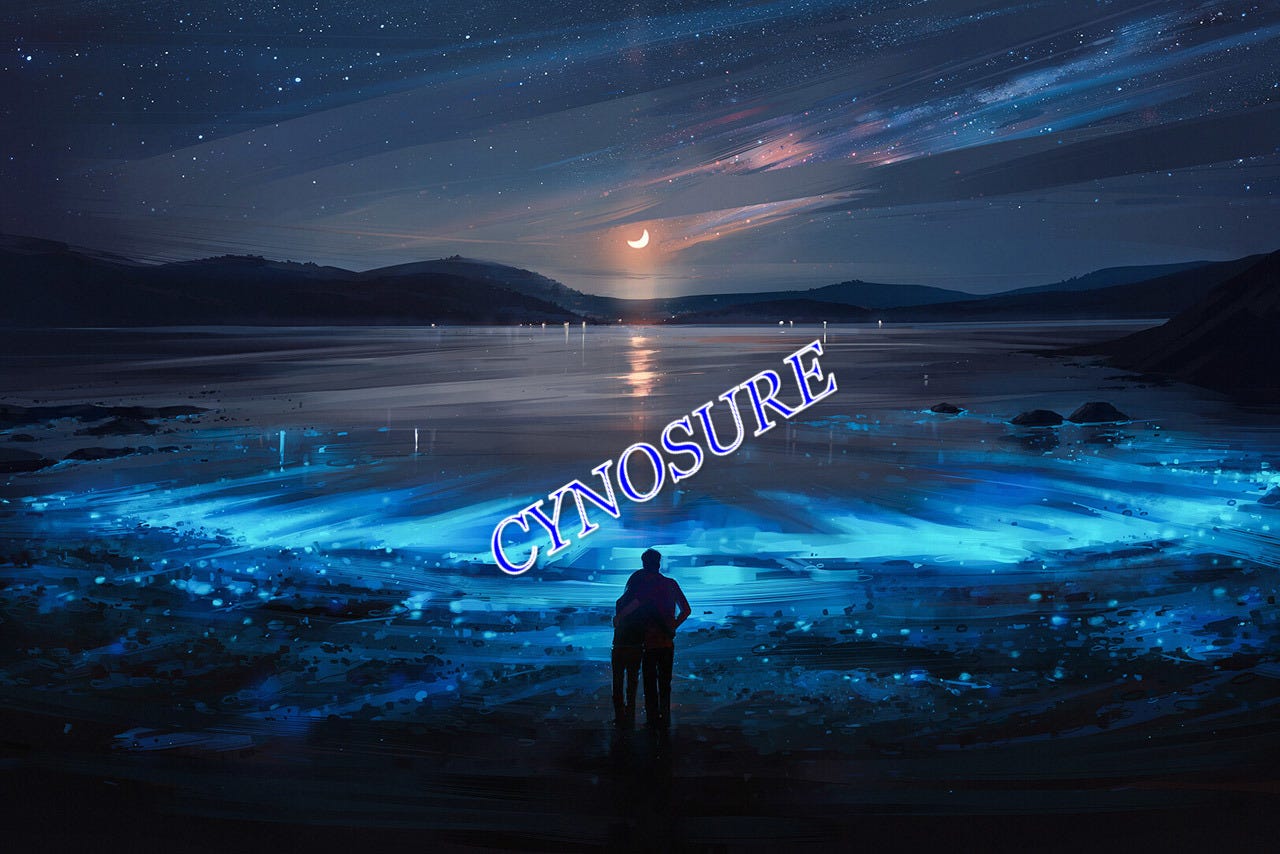The image depicts a serene and enchanting night scene, likely an illustration or graphic art, featuring a couple— a tall man and a woman—standing on a beach, embracing and gazing out over a breathtaking landscape. In the foreground, the beach glows with a bright blue light that contrasts beautifully against the dark, almost black background. Beyond the couple lies a body of water, shimmering under the light, and behind that, distant mountains add to the depth of the scene. The night sky is a canvas of various hues, with patches of blue and gray tones interspersed. Stars twinkle predominantly in the upper left corner, and a crescent moon, described as half-banana shaped, sits prominently near the center-right of the image, surrounded by a faint pink aura. The sky itself shows an artistic blend of colors, enhancing the dreamlike atmosphere. In purple uppercase letters, the word "CYNOSURE" is displayed across the middle of the image, hinting at the focal point or central theme of the artwork.